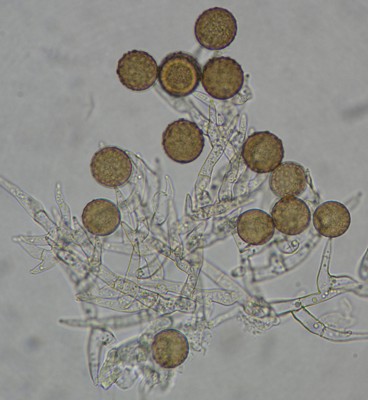This image appears to be a microscopic view of an unknown sample. The background features an off-white to light gray hue. Scattered across this backdrop are several almost round, brownish areas that could potentially be cells, eggs, or spores from an unknown organism. Additionally, the image showcases clear, elongated structures that are intertwined, centrally positioned. While these transparent structures have discernible borders, their exact nature remains unclear. The sample could represent biological material such as bacteria, plant matter, or parasitic elements, but the precise identification of these observed subjects is undetermined without further context.